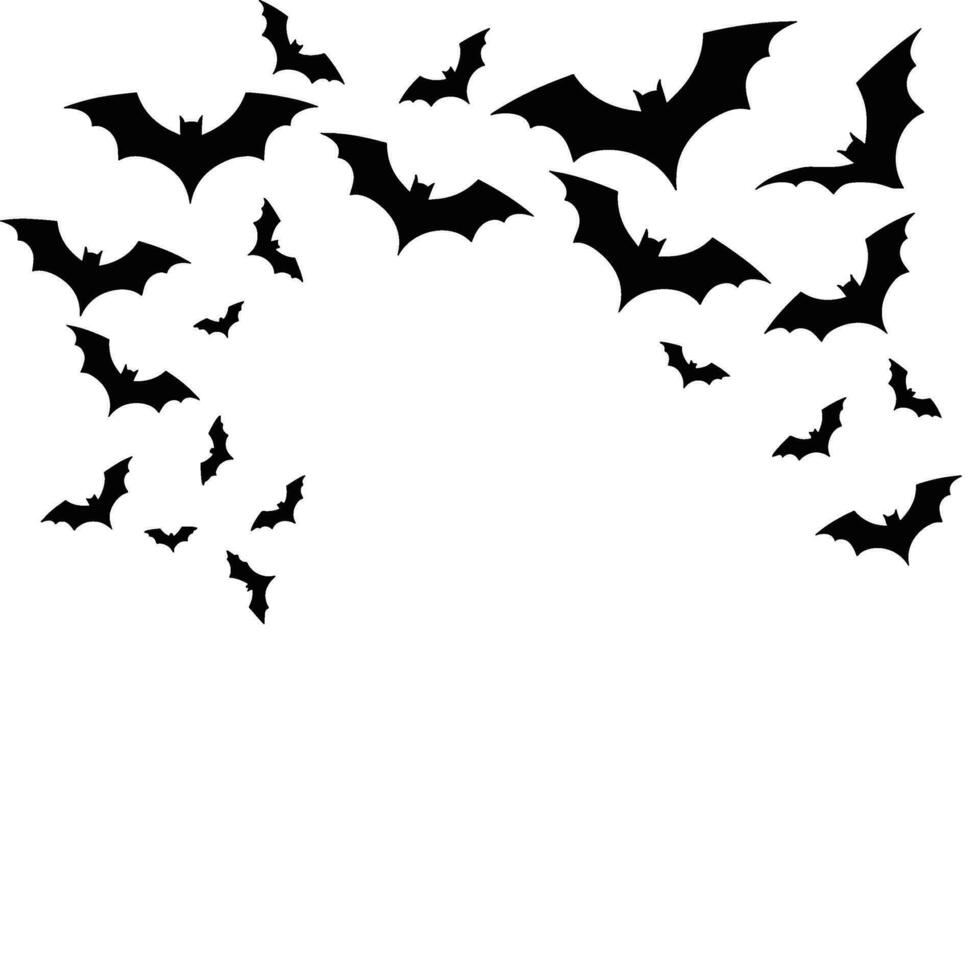The image features an intricate illustration of black bat silhouettes set against a stark white background. At least 50 bats of varying sizes are depicted, collectively forming an arch that stretches from the bottom left corner, ascends towards the top, and then descends to the right-hand side of the page. The repetition of the same bat image, varying in size to suggest depth and distance, creates a dynamic scene. Larger bats predominantly occupy the upper sections, particularly the top right and left areas, while smaller bats are more commonly found toward the bottom, interspersed with medium-sized ones. Each bat is in a different position, with some flying straight and others angled to the left or right, enhancing the sense of motion and chaos. There is no text or additional elements in the image, allowing the focus to remain solely on the bats that seem to float on the page without any defined border.